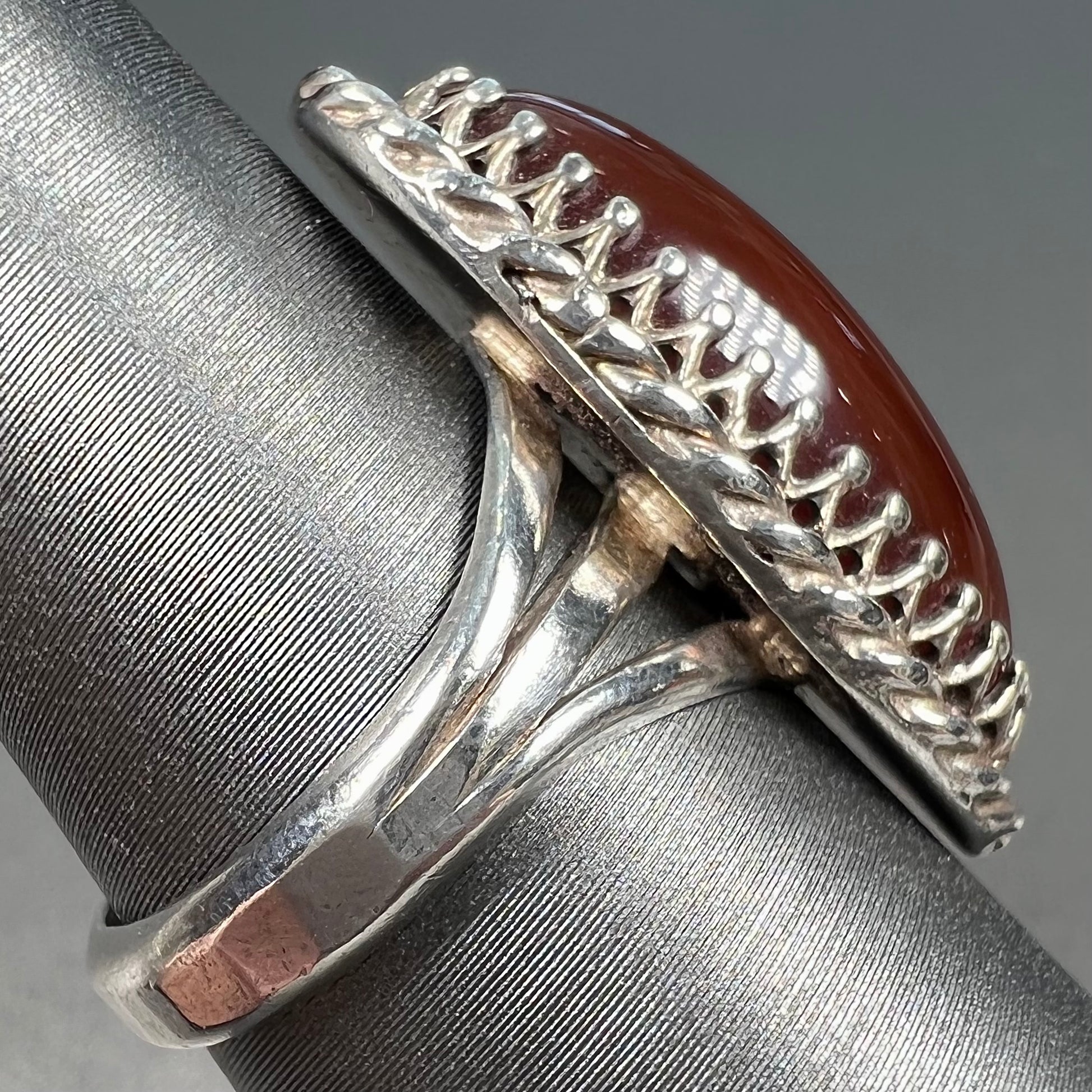The close-up color photograph showcases a striking silver ring mounted on a tapered, cone-shaped gray ring holder. The holder occupies most of the lower part of the image, gradually narrowing as it extends toward the top left corner. This silver ring features intricate welding with three stems at its base, and displays subtle gold-toned weld marks where the ring parts connect. The centerpiece of the ring is an oval-shaped gemstone, which is a rich, cranberry or carnelian color. Its smooth, curved surface and pronged setting, adorned with tiny balls at the tips, catch and reflect light beautifully. The ring's band exhibits a braided silver design that encircles the entire gemstone, adding an extra layer of elegance to the piece.